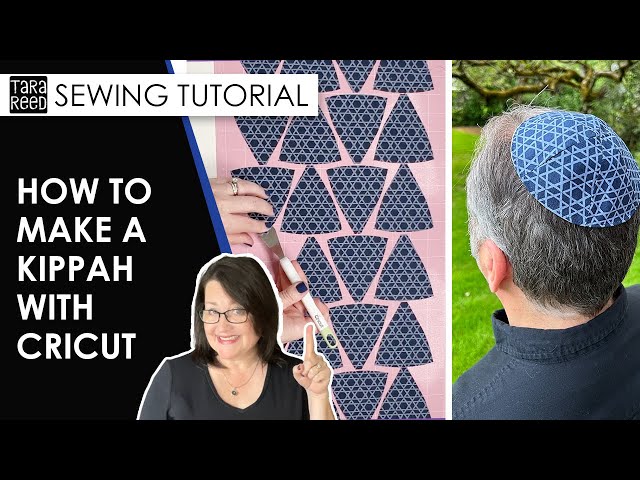The image is a detailed screenshot from a video tutorial titled "Tara Reads Sewing Tutorial: How to Make a Kippah with Cricut." The tutorial, presented by Tara Read, who is a woman with brown hair, glasses, a black shirt, and a small necklace, features her explaining and demonstrating the technique to create a Kippah, a traditional Jewish cap. The video overlay includes large white text on a black background indicating the title and subtitle. 

In the center, there's an image of a white fabric with blue triangular patterns, likely the fabric used to make the Kippah. A prominent picture shows a man with a combination of gray and dark hair wearing a Kippah. He is standing in a grassy area with a tree in the background, showcasing the final product. The bottom left corner of the image highlights Tara Read pointing up as she explains the steps. The borders of the image are framed with long horizontal black bars, adding a polished look to the presentation.